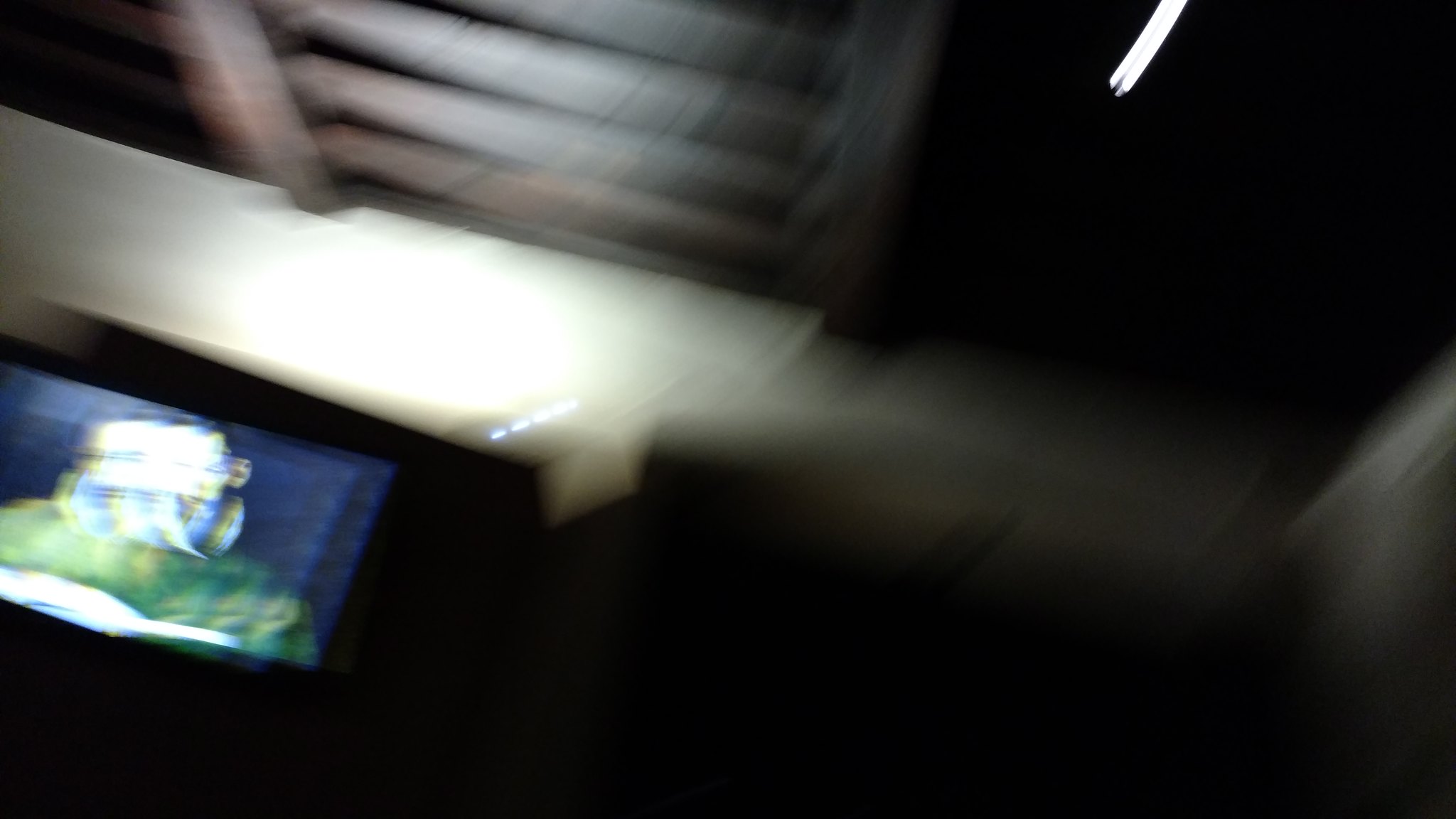This image is a very blurry, low-quality shot taken in a dimly lit room, likely resulting from camera movement. It appears to capture a TV or monitor screen positioned in the lower left corner, which depicts a person wearing a green shirt against a blue background. The person on the screen seems to have glasses and a beard. Above the display, there is a beige-colored wall illuminated by light, and the ceiling, which is black, includes visible rafters or beams. The image evokes a sense of motion due to the directional blur, suggesting the photo was taken while the camera was being moved or put down. Overall, the combination of poor lighting and motion blur obscures much of the detail in the photo.